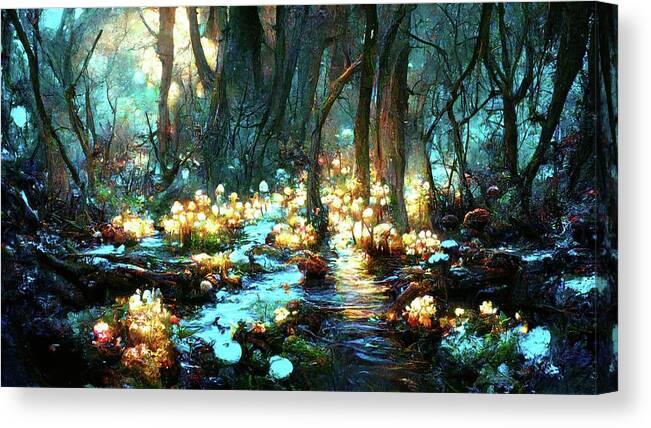This image vividly depicts an enchanted, dreamlike forest landscape at nighttime, masterfully captured in an impressionist painting on a canvas. The scene presents a surreal, almost mythical environment illuminated by vibrant, neon colors. The forest floor is adorned with clumps of luminescent mushrooms that glow in hues of blue, red, yellow, and pink, reminiscent of an ethereal fairyland. These glowing clusters create an enchanting atmosphere that extends throughout the image. The artist employs broad, expressive brushstrokes that give the painting a Monet-like quality, further enhancing its fantastical impression.

The background features a forest devoid of leaves, suggesting a wintry setting with bare brown trees. Interspersed between the trees are patches of natural light and eerie blue neon light, adding depth and a dreamlike quality to the scene. The ground appears slightly watery, contributing to the overall swamp-like ambiance. The combination of dark blues, purples, greens, and browns along with the luminescent colors creates a striking contrast, emphasizing the magical and surreal nature of this enchanted forest.